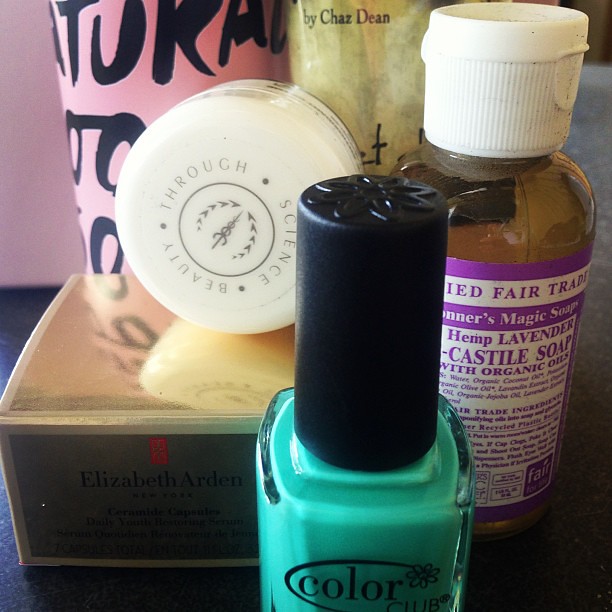The photo depicts an assortment of beauty products neatly arranged, likely on a table or shelf. Front and center is a vibrant, bright teal-colored nail polish bottle from Color Club. Directly adjacent to it is a clear bottle filled with golden liquid labeled as Hemp Lavender Castile Soap, featuring a white flip-top cap. To the left, there's a round bar of soap branded Thorough Scented Beauty and a box that says Elizabeth Arden, likely for a face cream or mask, with a smaller jar on top inscribed with 'beauty through science.'

Behind these items are two taller bottles: one yellow labeled by Shaz Dean and another in baby pink with black writing, displaying the letters T.U.K.A. Additionally, the setup includes other minor products like a brochure or sheet and possibly an instruction manual, adding to the overall detailed collection of high-end cosmetic and beauty items.